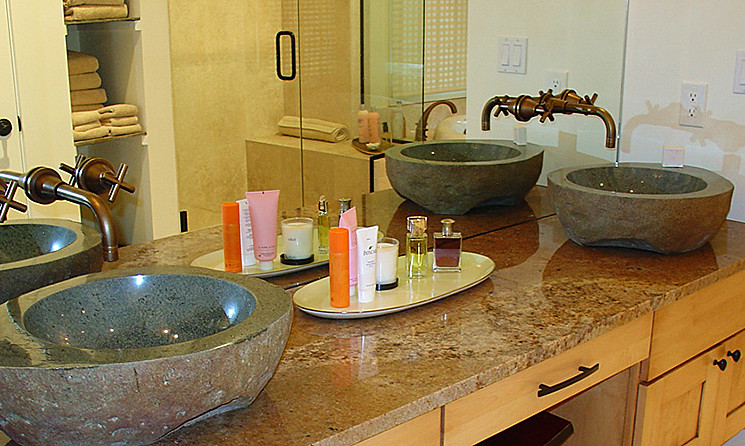This photograph showcases a contemporary bathroom featuring a sleek granite or marble countertop, approximately an inch thick, in various shades of brown with intricate striations. Below the countertop, the blonde wood cabinetry is contrasted by modern black handles, creating a stylish aesthetic. A full-length mirror spans across the back of the countertop, enhancing the room's sense of space. To the right, a white tiled wall houses an electrical outlet and a pair of light switches, which are visible in the mirror's reflection.

Prominently displayed on the countertop are two substantial stone sinks, distinguished by their thick, rugged, and unpolished rims, measuring at least three inches. The copper faucets, uniquely mounted directly into the mirror, add an elegant and innovative touch to the bathroom's design.